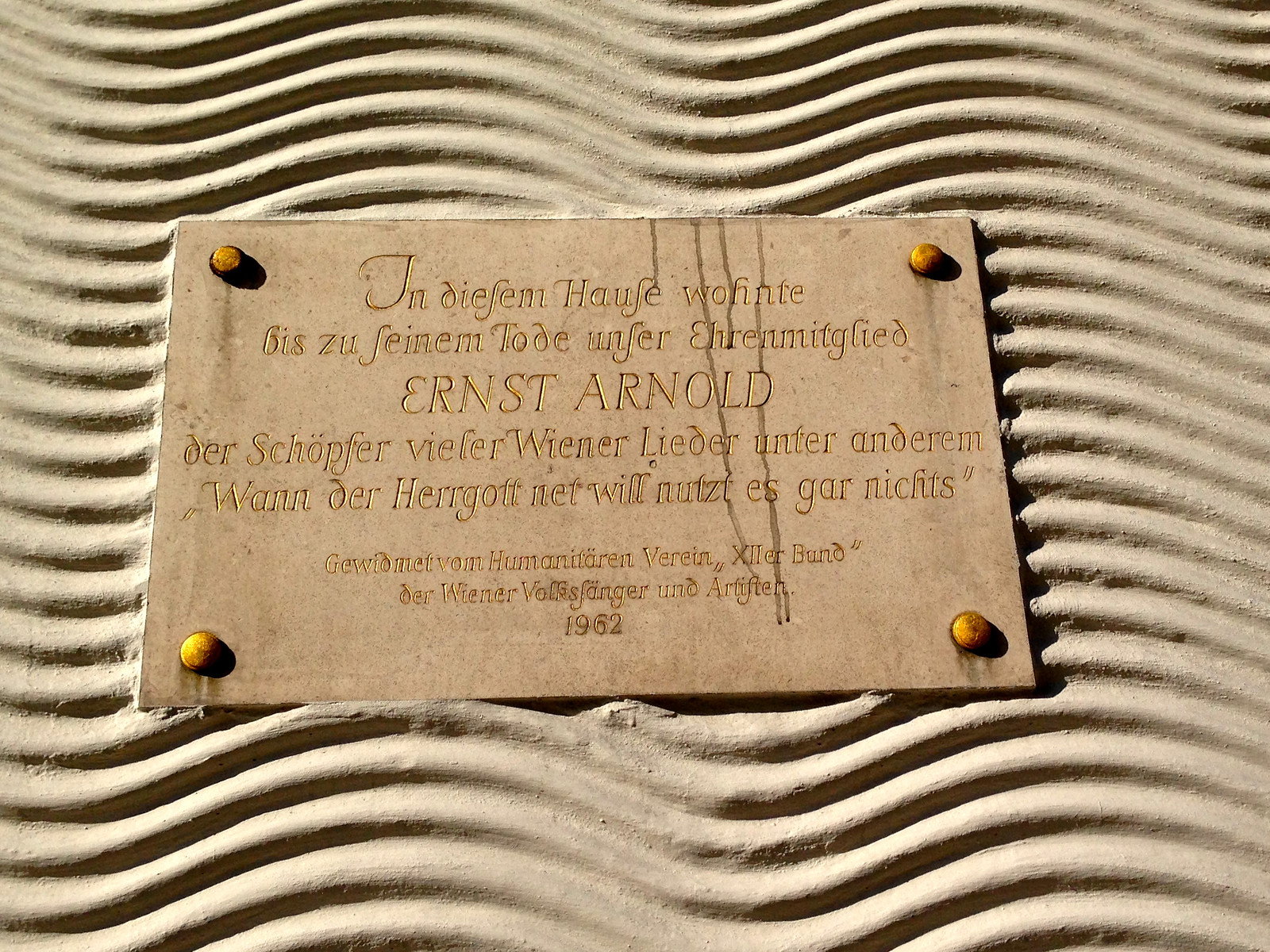This image features an aged, rectangular plaque that appears to be composed of a worn, tannish material. The plaque is mounted onto a lighter, wavy, indented background that looks like it could be made of cement or ceramic. The surface of the plaque is textured and shows signs of wear, with some water stains visible dripping from the top right corner. In the middle of the plaque, the name "Ernst Arnold" is prominently displayed in capital letters, surrounded by text in what is most likely German, written in an elegant, calligraphic golden font. The plaque is secured by three circular, gold-colored bolts, one in each corner, which have become rusted over time. At the bottom center, the date "1962" is clearly visible. This appears to serve as a memorial or tribute to Ernst Arnold.